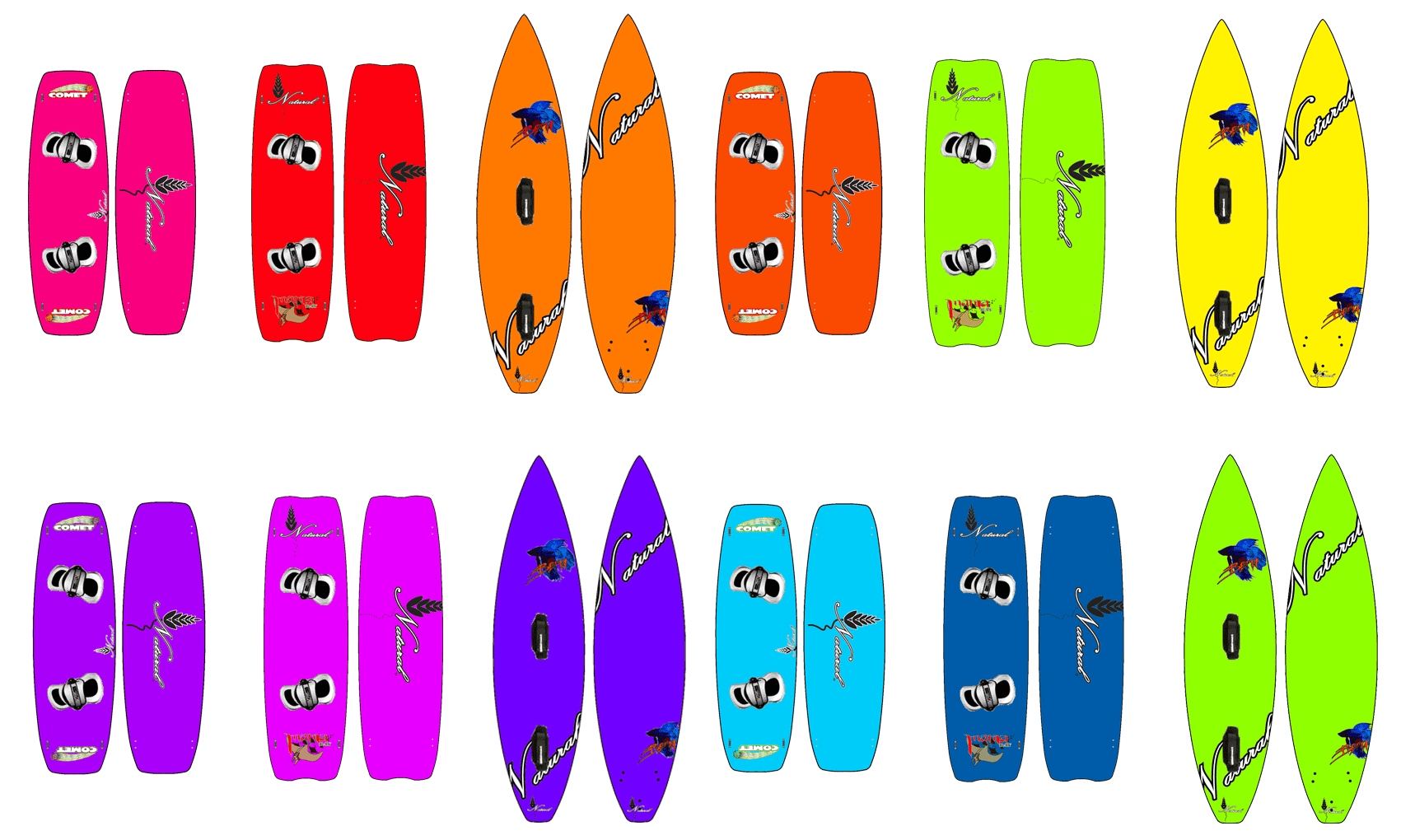The image is a detailed color illustration featuring two rows of various boards, each row showcasing six pairs of both surfboards and snowboards, depicted from multiple angles including front and back views. The boards are arranged in vibrant colors: from the top left, there is a pink snowboard, a red snowboard, an orange surfboard, a deeper orange snowboard, a green surfboard, and a yellow surfboard. On the bottom row from left to right, there is a dark purple snowboard, a violet snowboard, a lavender snowboard, a light blue snowboard, a blue snowboard, and another green surfboard. The snowboards are identifiable by the bindings for boots, while the surfboards (or possibly sailboards) have flat edges and foot platforms. Some boards feature logos and symbols, enhancing their distinctiveness. The background of the graphic is white, highlighting the vividness of the different colored boards.